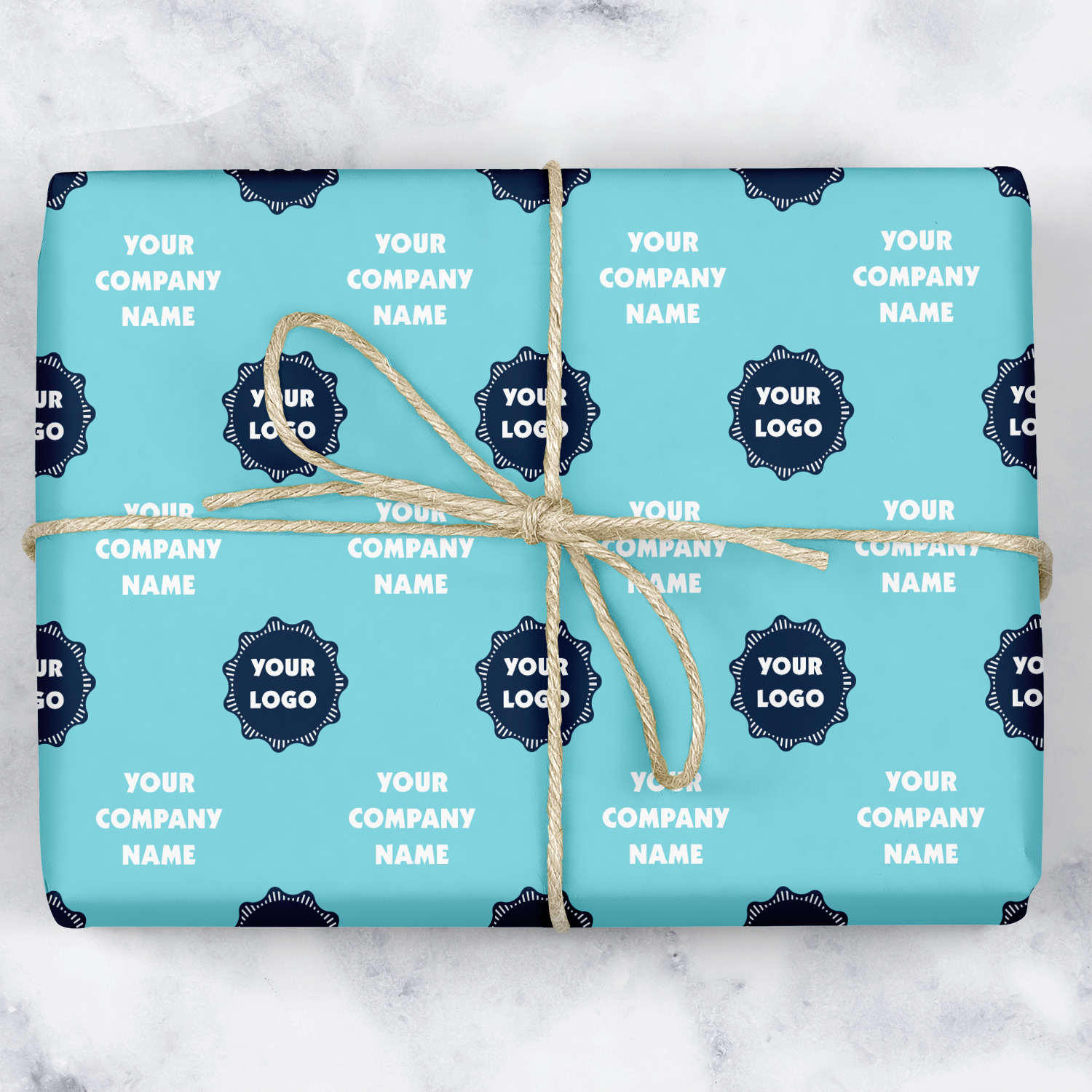The image depicts a promotional package from a custom gift wrapping company, showcasing their personalized wrapping service. The rectangular package is wrapped in light blue paper adorned with dark blue seals that feature the text "your logo" in white. These seals are arranged in four rows, with approximately five seals per row. Interspersed between the seals are three rows of the text "your company name," also in white. The entire package is neatly secured with an off-white twine bow that crosses the package horizontally and vertically, meeting in the center. The package is set against a light gray or white marble background, featuring subtle dark gray marbling, enhancing the visibility and elegance of the wrapping design.